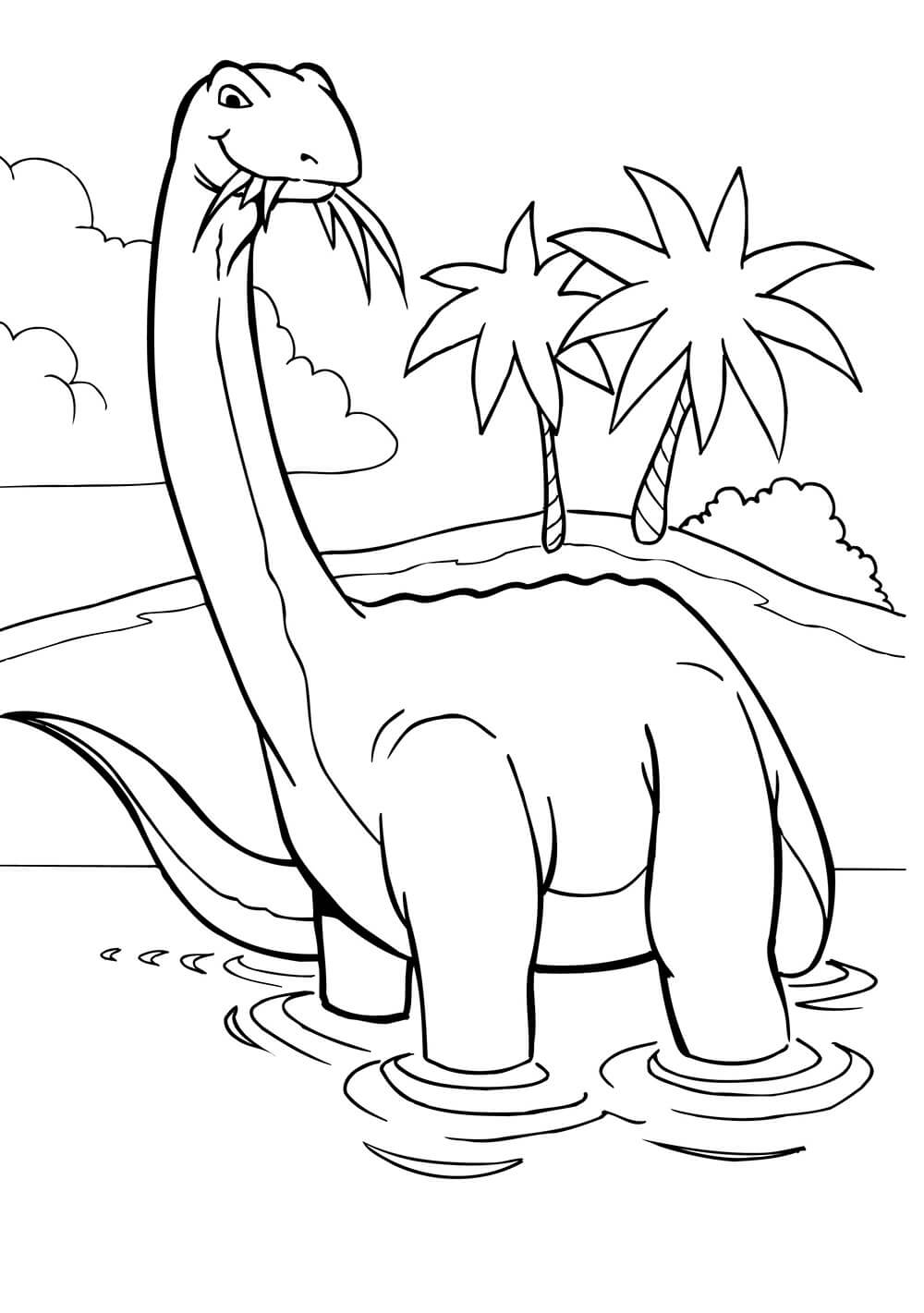The image resembles a child's coloring book page, delineated in black and white. It features a Brontosaurus-type dinosaur with a long neck and tail standing in a pool of water, causing ripples around its legs. The dinosaur is smiling and munching on some plants, with its head turned towards the viewer. The background showcases a small, hump-shaped island with two palm trees and some brush at its base. A large, puffy cloud occupies the left side of the sky, further enhancing the whimsical scene. The minimalist style, reminiscent of a cartoon, invites coloring and fills the image with a playful and inviting atmosphere.